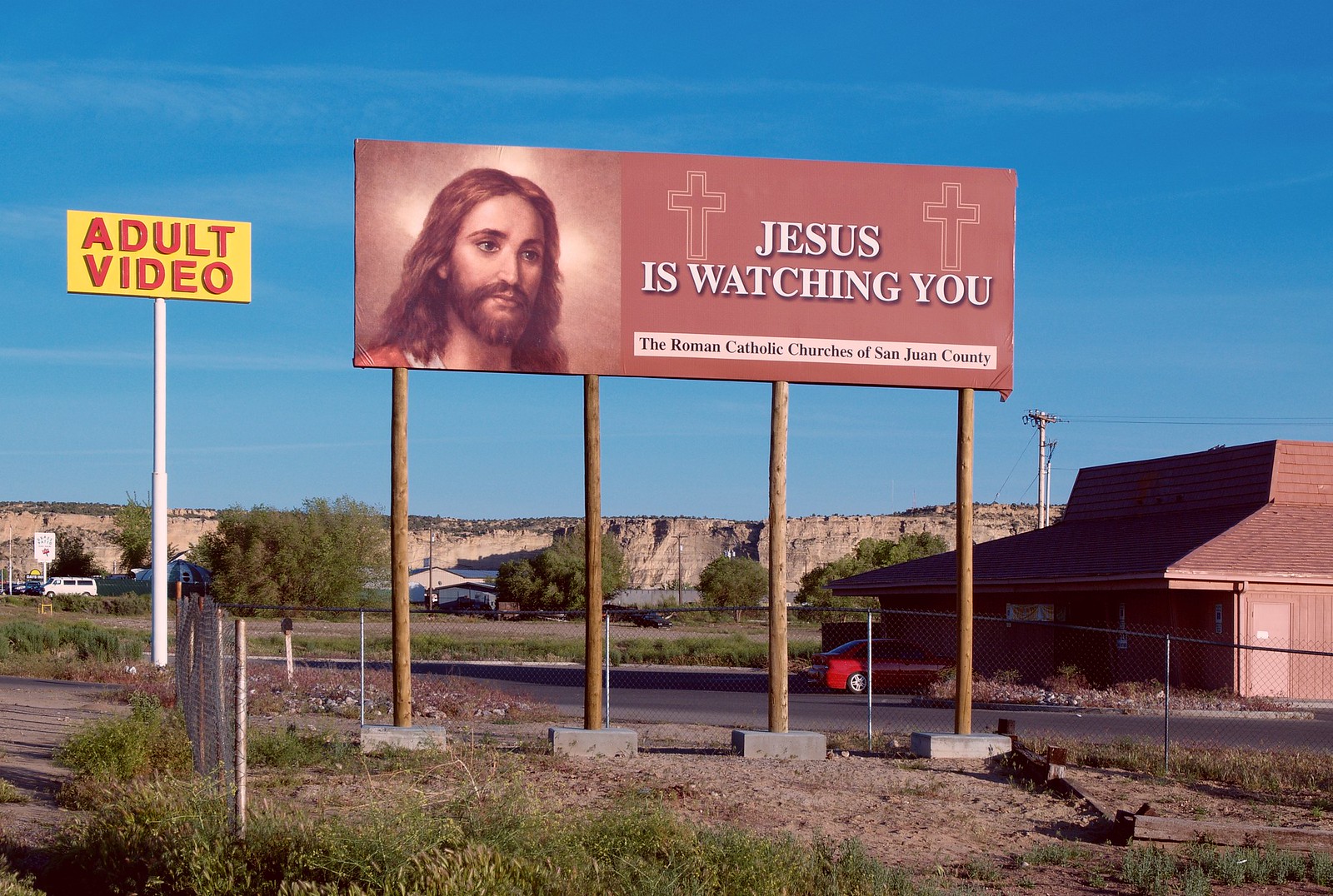The photograph depicts an outdoor scene dominated by two billboards amidst an arid, desert-like landscape with a few buildings and cars visible. In the center, a prominent light reddish billboard, supported by four wooden poles standing on a chain-link fence foundation, features an image of Jesus Christ with long hair and a beard. Beside two crosses on the billboard, the text boldly declares, "Jesus is watching you," followed by a white rectangle beneath that states, "The Roman Catholic Churches of San Juan County." To the left of this billboard, a smaller sign on a long white pole displays the words "adult video" in bold red letters against a yellow background. Behind these signs, a few scattered buildings, including a red-roofed structure, are visible, along with a red car. The background is completed by barren hills or cliffs under a vibrant blue sky, giving the area a somewhat desolate yet striking appearance.